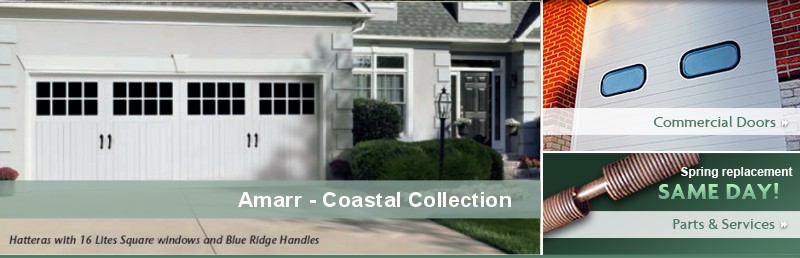This advertisement, rectangular in shape and divided into two sections, showcases two distinct products. The larger left section features a grey house with a double garage door. Each door has 16 black window panels, totaling 32 panels, arranged in two rows to simulate the appearance of individual glass panes. The double garage doors, designed to open in the middle, have two black handles each. In the bottom right corner of this section, text reads "Amar Coastal Collection" in white, while the lower left corner has details about the doors: "Hatteras with 16 lights square windows and blue ridge handles." The house is further described with shrubs adorning its front yard, a front window, a glass door, and a grey roof.

To the right, the smaller square section highlights another product: a commercial door. This white slide-down door is set in a brick building, featuring two blue oval-shaped windows. A banner across the door reads "Commercial Doors." Below this image, there is a segment dedicated to spring replacement services. A copper coil spring is displayed, accompanied by the text "Spring Replacement" in bold white letters on a green background. The phrase "Same Day!" is emphasized in bolder green letters, with "Parts and Services" mentioned in less bold green letters, all set against a white background.